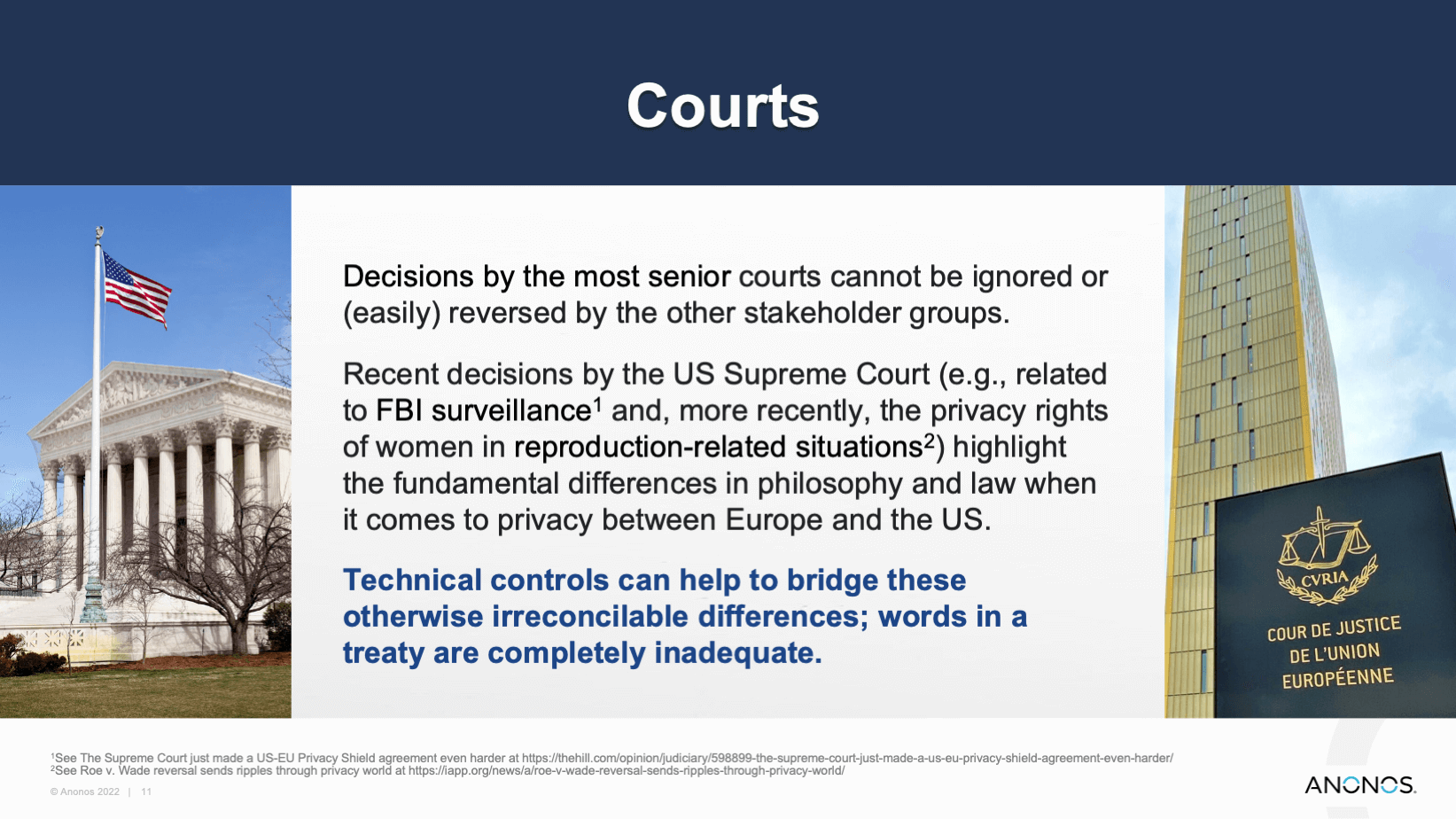The webpage features an article focused on judicial systems, predominantly comparing the US and European courts. At the top of the screen, a dark blue bar displays the word "courts" in white text. 

On the left side, there's an image of the US Supreme Court building, basking in bright sunshine on a winter day, as evidenced by the leafless trees. An American flag stands at full mast beside the court.

To the right, another image showcases a tall building with distinctive yellow and white patterning and windows. It also includes a golden-embossed placard, which resembles a passport, bearing the label "CVRIA" and the scales of justice. The inscription reads "Cour de justice de l'Union européenne," indicating it is the European Court of Justice.

Centrally placed between these images is a block of text discussing notable decisions made by senior courts. It mentions recent rulings by the US Supreme Court, such as those related to FBI surveillance and women's privacy rights concerning reproductive matters. These cases underscore the stark contrasts in privacy philosophies and laws between Europe and the US. Highlighted in blue text, the narrative suggests that technical controls could help reconcile these differences, as mere treaty words are deemed inadequate.

At the bottom of the text, references are provided:
1. "The Supreme Court Just Made a US-EU Privacy Shield Agreement Even Harder" from The Hill (URL: http://thehill.com/opinion/judiciary/598899-the-supreme-court-just-made-a-us-eu-privacy-shield-agreement-even-harder).
2. "Roe vs. Wade Reversal Sends Ripples Through Privacy World" from IAPP (URL: https://iapp.org/news/a/roe-v-wade-reversal-sends-ripples-through-privacy-world).

The content is published by Anonos, marked with a copyright notice for the year 2022.

This detailed webpage commentary contrasts the judicial landscapes of the US and Europe, emphasizing current events and the potential for technological solutions in bridging legal disparities.